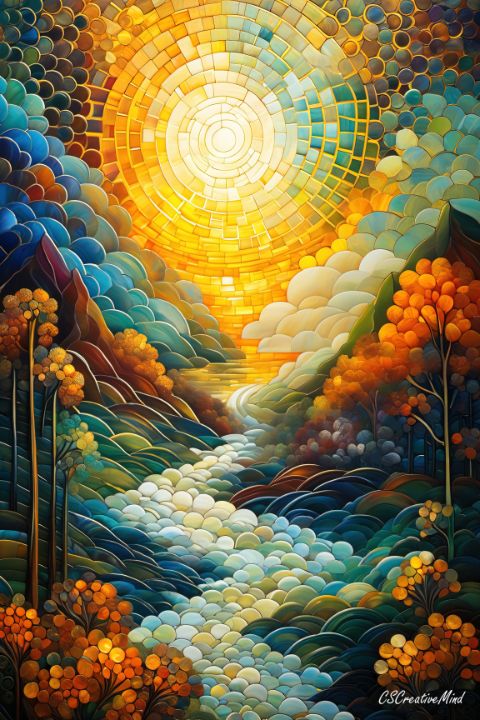This painting, rendered in a vertical rectangle, combines a vibrant array of circles and squares to create an abstract yet discernible landscape. Dominating the top center, a sun composed of square tiles features a bright white core encircled by layers that transition from yellow to orange, finally blending into light blue and green hues toward the top right. On either side of the sun, the image depicts blue and white circular forms, contributing to a sense of atmospheric depth, potentially representing clouds. Below the sun, a dynamic river meanders in a zigzag pattern through the valley, filled with white, light blue, and pale green circles, lending a reflective quality to the water. Flanking the river, jagged, brown, and green mountains rise, appearing wavy and textured. Tree branches with clusters of orange circles, resembling flowers or foliage, emerge on both the left and right sides of the picture, adding to the naturalistic elements. These orange circles also appear as shrubs or bushes near the bottom of the riverbanks. The entire scene, intricately detailed, uses varying sizes and colors of circles and squares, creating a textured, almost mosaic-like interpretation of a sunlit valley with a flowing creek and surrounding mountainous terrain. In the bottom right corner, a small white signature is visible, though difficult to decipher.